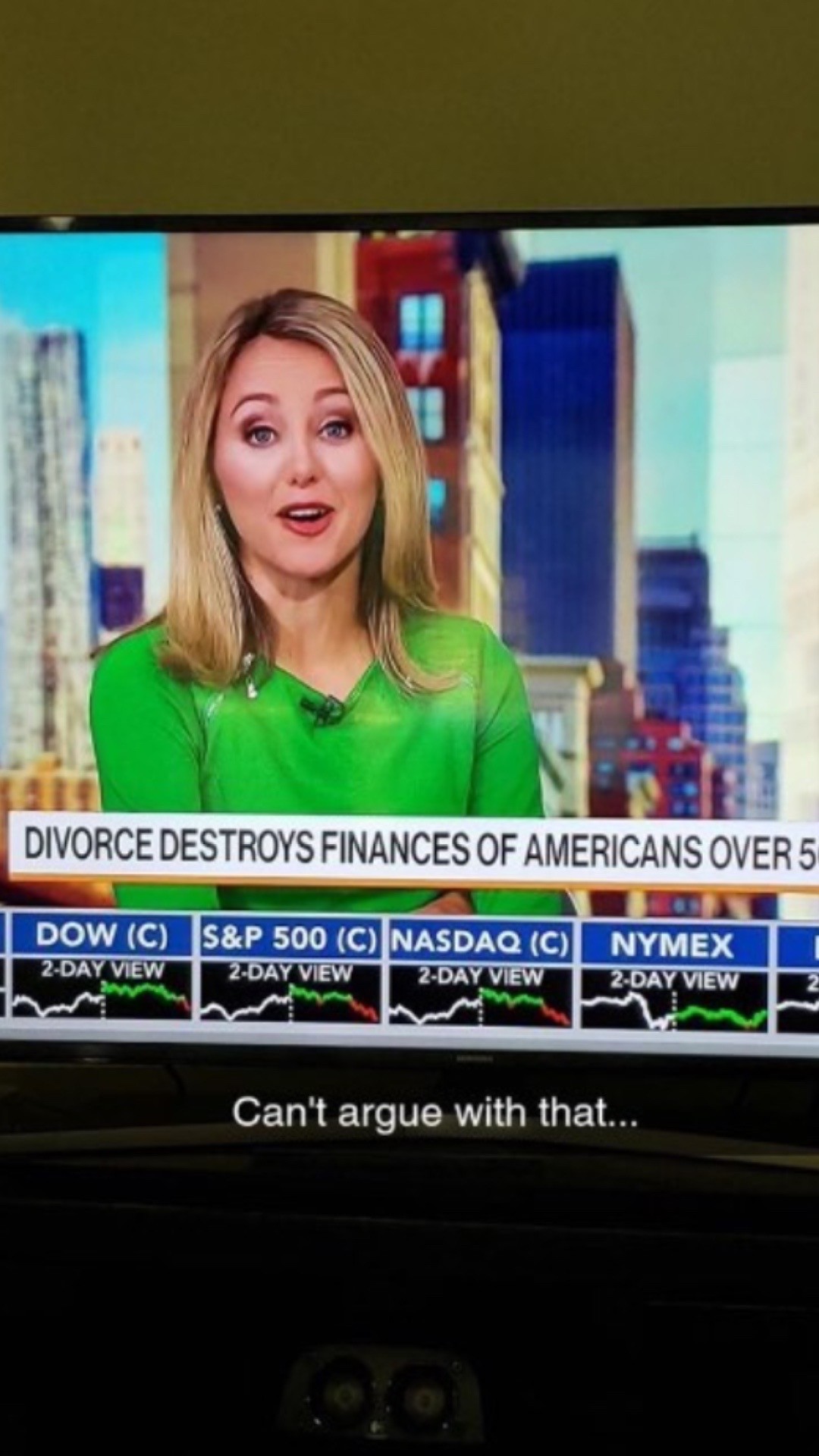A photograph captures a dimly lit TV screen showing a female news anchor in a portrait orientation. The anchor, a white woman with shoulder-length, slightly flared blonde hair, is wearing a green blouse. Behind her, there is a nondescript cityscape featuring several buildings. At the bottom of the screen, a stock market ticker displays the Dow, the S&P 500, the NASDAQ, and NYMEX two-day view charts. A headline on the ticker reads, "Divorce Destroys Finances of Americans Over 5," with the rest of the number cut off, likely intended to signify "50" or "55." Below this, a caption in smaller text states, "Can't Argue With That..." The photograph appears to have been taken by someone capturing the image off their TV screen, and in the lower dark section of the image, there seem to be dim eyeballs and a head subtly visible, peering out.